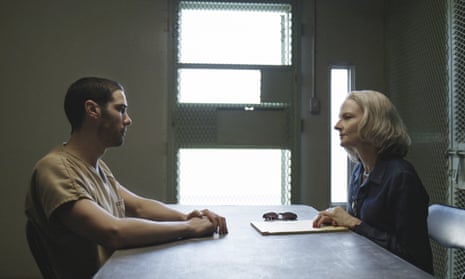The image, a smooth and possibly digitally enhanced artwork, portrays a tense and serious scene that resembles an interrogation or an interview. Set in a sparse, drab room with light tan walls and backlit by four distinct windows or a large glass door that adds to the somber atmosphere, the composition centers on two individuals seated at a long, dark metal table with metal chairs. On the left side sits a young man with dark hair, donned in a plain brown short-sleeved shirt, reminiscent of a prison uniform. Opposite him, on the right, is a blonde woman in a dark suit, likely an investigator or lawyer, who has a manila folder or tablet and sunglasses laid out in front of her. Both figures are serious, with the woman’s hands resting on her folder and the man leaning slightly forward, their eyes locked in a moment of intense, silent communication.